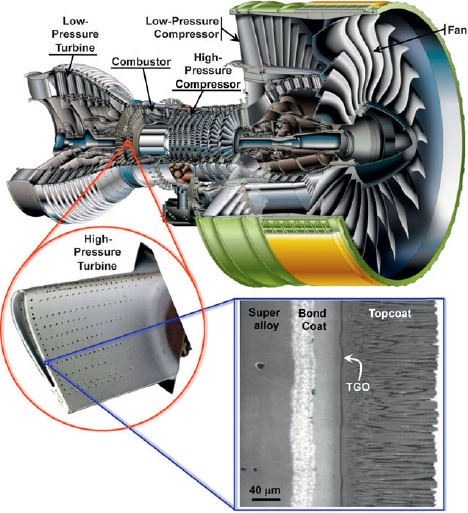This image is a detailed cross-sectional diagram, likely from an educational brochure or an owner's manual, depicting the internal components of an engine. The diagram, primarily rendered in black and white, showcases a series of intricate parts, including multiple gears and fans, arranged sequentially from left to right.

On the far left, labeled components include the low-pressure compressor and the high-pressure compressor, followed by the combustor. Subsequent elements feature the low-pressure turbine and at the far right, a highlighted fan encased within a green and yellow tubular structure. This rightmost section draws particular attention due to its colorful distinction.

Central to the diagram is a red-circled, close-up view of a high-pressure turbine located on the lower left-hand side, with an even more detailed inset at the bottom right. This high-pressure turbine is described with annotations indicating construction materials such as super alloy, bond coat, and top coat. An arrow points to a labeled subsection denoted as "TGO."

The illustration serves to provide a clear understanding of the internal mechanics, emphasizing the layered complexity and specific material composition of engine components, particularly the high-pressure turbine.